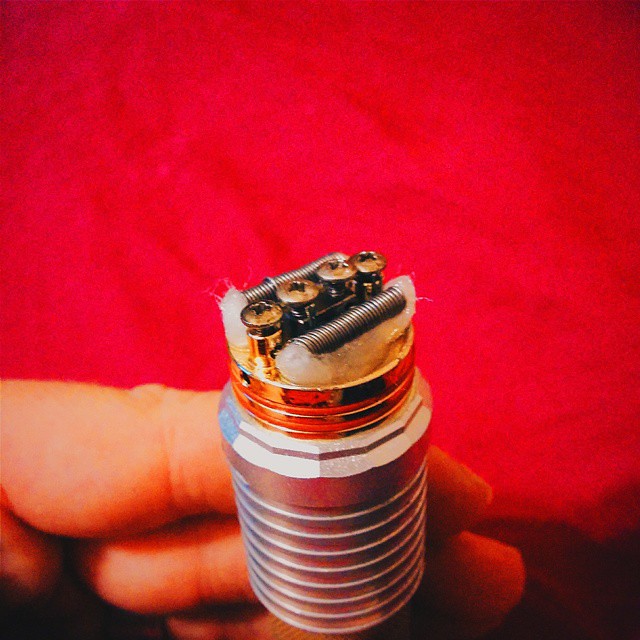This is an image of a small, intricate mechanical object held by a fair-skinned hand against a red background. The object is a cylindrical metallic structure, primarily silver with a golden top. It has multiple layered sections, with the top layer being the thickest. At the top, there are four Phillips head screws embedded in the gold section. Next to these screws are two metal coils, each with a white cotton-like material emerging from them. The entire assembly is compact, only occupying the tips of the person's fingers. The background is a consistent red, suggesting either a bed sheet or some other fabric surface.